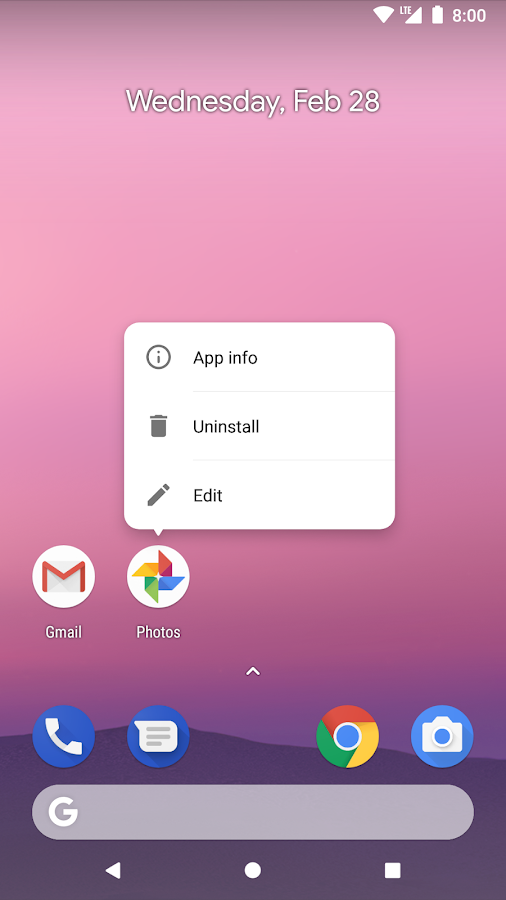This image captures a screenshot of an Android smartphone's home screen with a distinct pink background. In the top right corner, icons display important status information: a strong Wi-Fi connection, full signal strength, a fully charged battery, and the current time, 8:00 AM. Centered at the top of the screen, the date reads "Wednesday, February 28th."

The home screen features six icons arranged in two rows:
1. Gmail
2. Photos (selected, indicated by a responsive options box showing "App info," "Uninstall," and "Edit")
3. Phone
4. Messaging (text messaging)
5. Google Chrome
6. Camera

Beneath these icons, a Google search bar is prominently placed, identified by its gray background and the white letter "G." 

At the bottom of the screen, standard navigation buttons of an Android device are visible:
- The Back button on the left
- The Home button in the center
- The square button for the app drawer on the right.